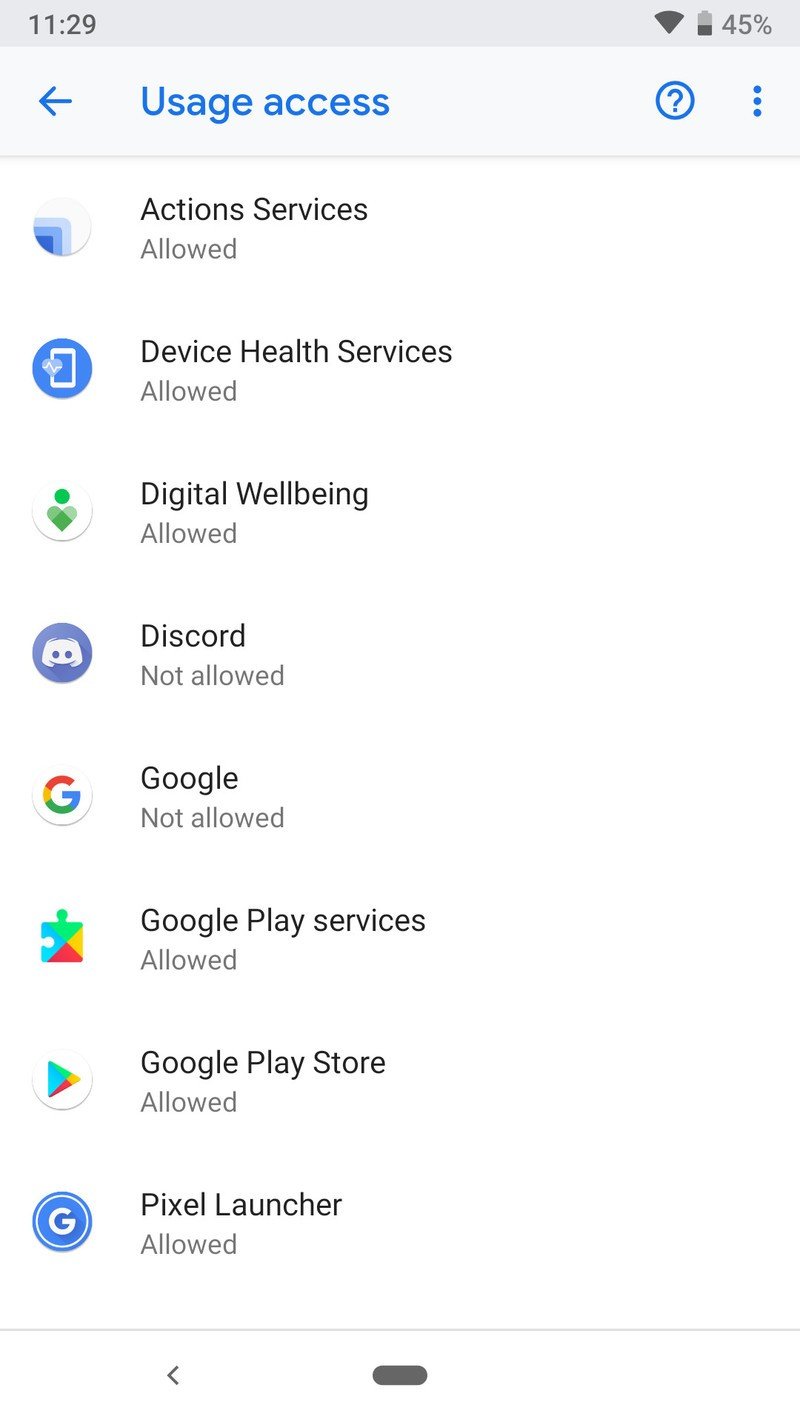Detailed screen capture of a cell phone at 11:29 AM with 45% battery. The status bar shows a full internet connection. The screen is displaying a "Usage Access" settings menu, indicated by a back button option and a three-dot menu for additional settings.

Listed services and apps with corresponding icons include:
1. **Action Services** - Allowed
2. **Device Health Services** - Allowed, marked by a blue icon.
3. **Digital Well-being** - Allowed, marked by a green icon.
4. **Discord** - Not allowed, marked by a light purple icon resembling a smiley face.
5. **Google** - Not allowed, marked by the Google "G".
6. **Google Play Services** - Allowed, marked by a puzzle piece icon.
7. **Google Play Store** - Allowed, marked by the Google Play symbol.
8. **Pixel Launcher** - Allowed, marked by a blue "G".

The screenshot provides a clear overview of the permissions set for various applications on the phone.